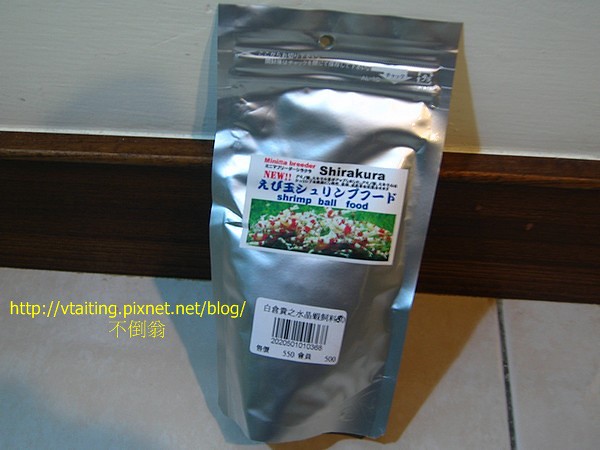This photograph captures a product package, likely positioned indoors, on a kitchen floor with a wooden baseboard along the bottom of the wall. The package is a shiny, silver pouch that stands out vividly against its surroundings, almost resembling an outer space silver. The pouch is leaning against the wall and is labeled with a white sticker at the top that reads "Shirakura" in black text and "shrimp ball food" below in blue text. The rest of the writing on the package is predominantly in Japanese.

The silver pouch also features a vibrant photo with a green background showcasing numerous red bits of food, presumably the shrimp balls. Above the photo, in bold red lettering, the word "NEW" is prominently displayed. Beneath this image, there's a barcode displayed on another white sticker labeled with the UPC code 20-20-50-10-10-3-6-6-5-50.

For those interested in purchasing the product or obtaining more information, a website address is provided on the lower left-hand corner of the pouch in yellow text: http://vtaing.fixnet.net.blog/.